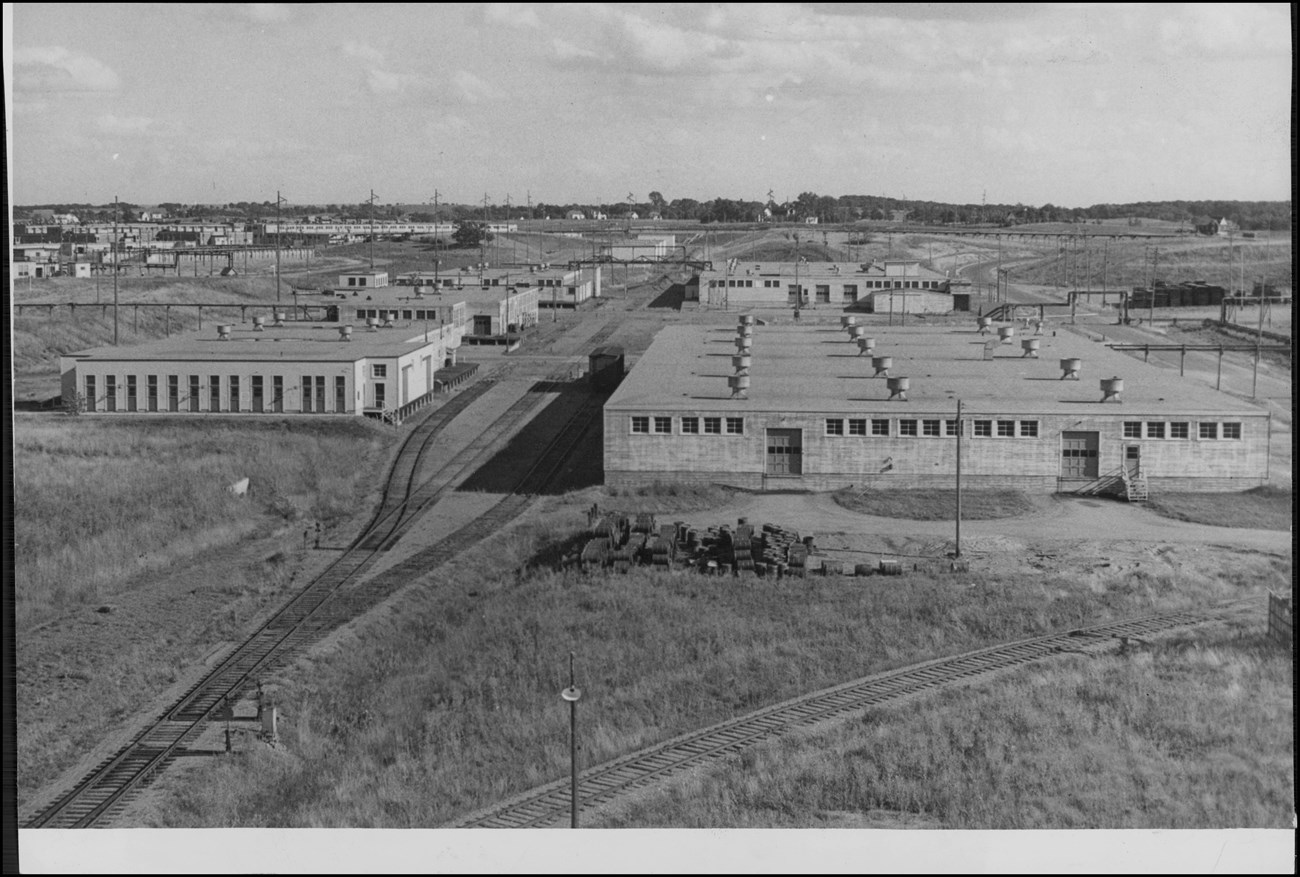A striking black and white photograph captures a tranquil yet mystifying scene. The sky above, lightly adorned with scattered clouds, descends gracefully to meet a distant tree-lined horizon. This serene backdrop is juxtaposed with an array of one-story buildings that stretch across the middle ground of the frame. Each structure, rectangular and uniformly flat-roofed, is punctuated by numerous small windows and occasional doors, presenting an organized, grid-like appearance. Parallel rows of these edifices create a corridor effect, enhanced by the presence of train tracks that intersect the area, with one prominent set curving off towards the right side of the image. The buildings, though industrial in design, lack clarity in their purpose, evoking an ambiguous ambience — neither entirely utilitarian nor comfortably familiar. The closest building to the viewer is notably large and rectangular, dominating the immediate foreground with its imposing presence. The entire composition, devoid of color, relies on the interplay of light and shadow to evoke a timeless, almost haunting atmosphere.